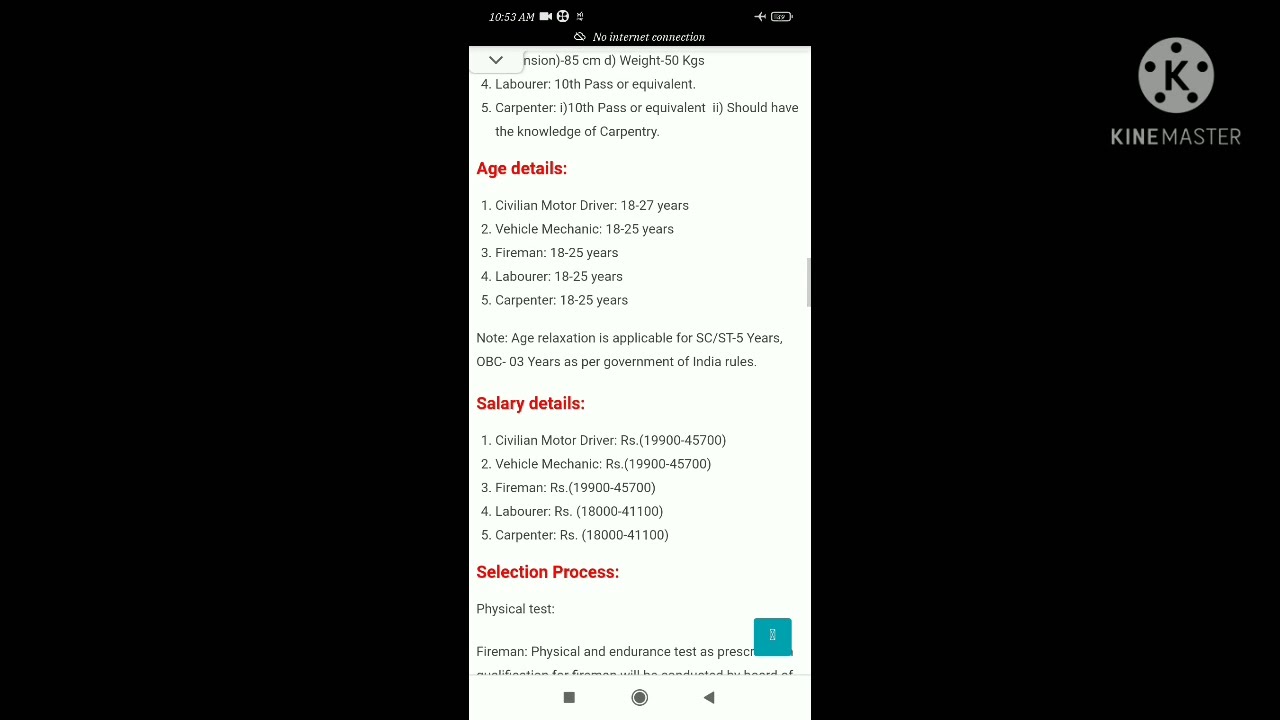The image is a screenshot from a phone displaying a detailed recruitment chart for various occupations. The chart, visible on a vertically rectangular white background, includes numbered lists, job titles, age requirements, and salary ranges. Around the content, there are black bars, indicating it was captured in landscape mode on a phone. In the top section, the phone’s interface shows a battery icon and airplane mode indicator. On the right, there is a white circle logo with five paper punches and a large letter "K", labeled "KineMaster."

The chart lists job titles such as Civilian Motor Driver (18 to 27 years old), Vehicle Mechanic (18 to 25), Fireman (18 to 25), Laborer (10th pass or equivalent, 18 to 25), and Carpenter (11th pass or equivalent, 18 to 25, should have knowledge of carpentry). There is an age relaxation note indicating a five-year extension for certain applicants. Salary details are provided, with typical salaries ranging from $19,900 to $45,700 annually for most jobs, with laborers and carpenters earning slightly less, from $18,000 to $41,000. The process for selection is mentioned, with a physical test required for each position. The screenshot highlights the underwhelming wages and specific criteria for each job role, likely sourced from a website providing detailed job-related information.